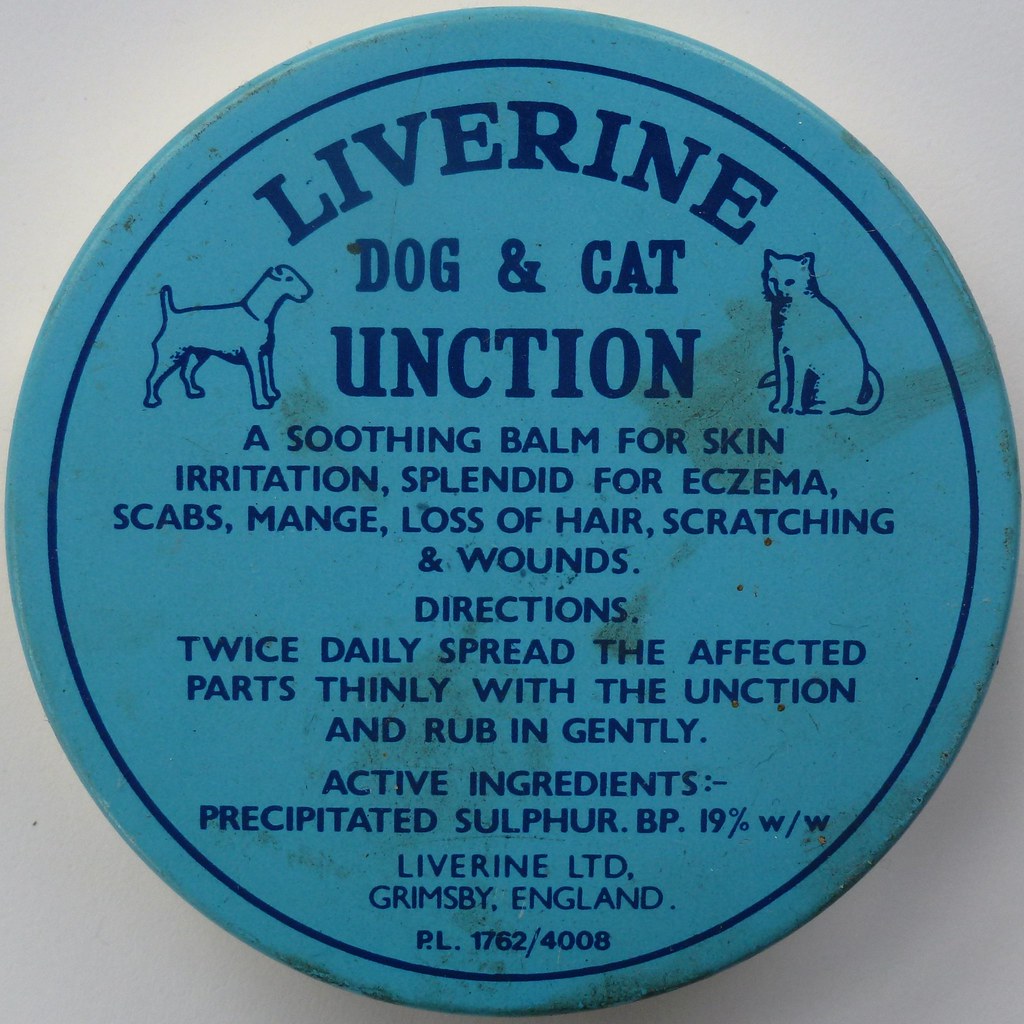The image depicts a worn, circular blue label that likely adorns a small canister or jar. The label features a darker blue circle inside a lighter teal-blue background. At the top, in concave, rounded text, it reads "Liverine." On the left side is a graphic illustration of a dog, while the right side shows a cat. Below the main title, the label states "Liverine Dog and Cat Unction," though it may intend to mean "function."

The label describes the product as "a soothing balm for skin irritation, splendid for eczema, scabs, mange, loss of hair, scratching, and wounds." Usage instructions indicate to "spread the affected parts thinly with the unction twice daily and rub in gently." The active ingredient is listed as precipitated sulfur at 19% BP, W/W. The label also provides details about the manufacturer: "Liverine Ltd, Grimsby, England, PL 1762/4008." The entire label is set against a white surface and shows signs of aging with some stains and wear.